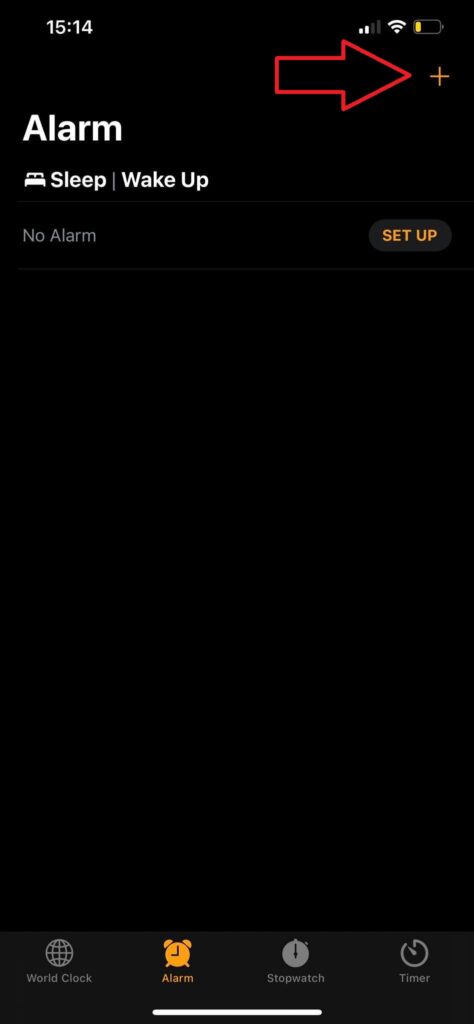The image is a screenshot of the Clock app on an iOS device, displayed in dark mode. It is vertically oriented, showing detailed information at the top such as the time (15:14), Wi-Fi signal strength, cellular network signal strength, and remaining battery life. The primary section of the image is focused on the Alarm tab, identifiable by the highlighted alarm clock icon at the bottom of the screen.

In the Alarm tab, the background is black, with text in white and yellow. The words "Alarm" and a small bed icon labeled "Sleep" appear prominently. Beneath these, a bar indicates "Wake Up," though no alarms have been set yet. To the right, a red arrow annotation points to a plus sign, suggesting how to add a new alarm. 

The screen also displays a "Set Up" option, indicating another method to configure an alarm. At the bottom menu, the available tabs include World Clock, Alarm (which is currently selected), Stopwatch, and Timer. Each of these tabs offers interactive buttons for navigation within the app. Users can either set up a new wake-up time by tapping the plus button or by selecting the "Set Up" option.